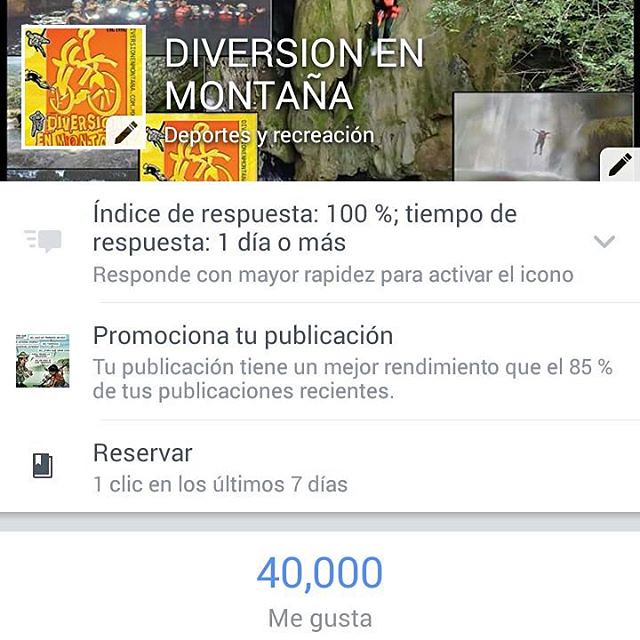This is a detailed color screenshot of a Spanish-language social media post, likely from Facebook, showcasing various outdoor recreational activities. At the top, the post features a banner with the heading "Diversión en Montaña" and "Deportes y Recreación" in white text, set against a vibrant backdrop. The banner includes a logo on the left, a yellow square with the black silhouette of a bicycle on an orange background. Alongside the logo, the text reads, “Diversión en Montaña,” with an accent over the 'ñ', emphasizing the theme of mountain fun and recreation.

The central section of the post is divided into smaller images. On the left, a person is seen rock climbing on a rugged wall, surrounded by dark green foliage, dressed in an orange and red suit. To the right, a smaller image captures someone in mid-air, leaping off a waterfall, with the cascading water and moss-covered rocks vividly depicted. There's also an image of a group of people in a cave, equipped with gear and lights, illustrating diverse adventures.

In terms of social media metrics, at the bottom of the post, we see the number "40,000" highlighted in blue next to the phrase "me gusta," indicating the post's popularity. Below this, a block of detailed Spanish text discusses the responsiveness and promotional aspects of the publication, including phrases like "Índice de respuesta: 100%," "Promêcia tu publicación," and “Tu publicación tiene un mejor rendimiento que el 85% de tus publicaciones recientes," stressing the post's high engagement and effective performance. The call to action "Reserva con un clic en los últimos 7 días" suggests booking activities within the last week.

This vibrant, multi-image advertisement invites viewers to partake in thrilling outdoor activities, all set in natural and adventurous locations.